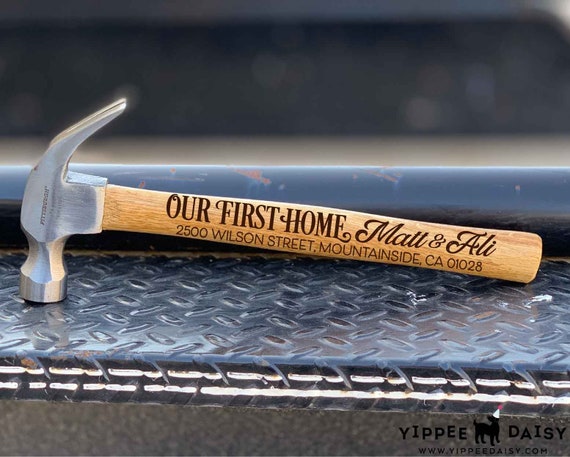This close-up outdoor daytime image captures a detailed view of a hammer resting on the back bumper of a truck. The hammer has a wooden handle and a shiny metal head. The handle features black, all-capital letters that read, "Our First Home, Matt and Allie, 2500 Wilson Street, Mountainside, California, 01028." The truck's bumper, located at the bottom of the picture, is silver with small ridges. The background reveals the rest of the truck, although it is out of focus. In the bottom right-hand corner of the image, the words "Yippee Daisy" are visible alongside a logo depicting a black dog with a white party hat adorned with a red pom-pom. This caption is accompanied by the URL www.yippeedaisy.com, suggesting that Yippee Daisy may be the producer associated with the hammer.